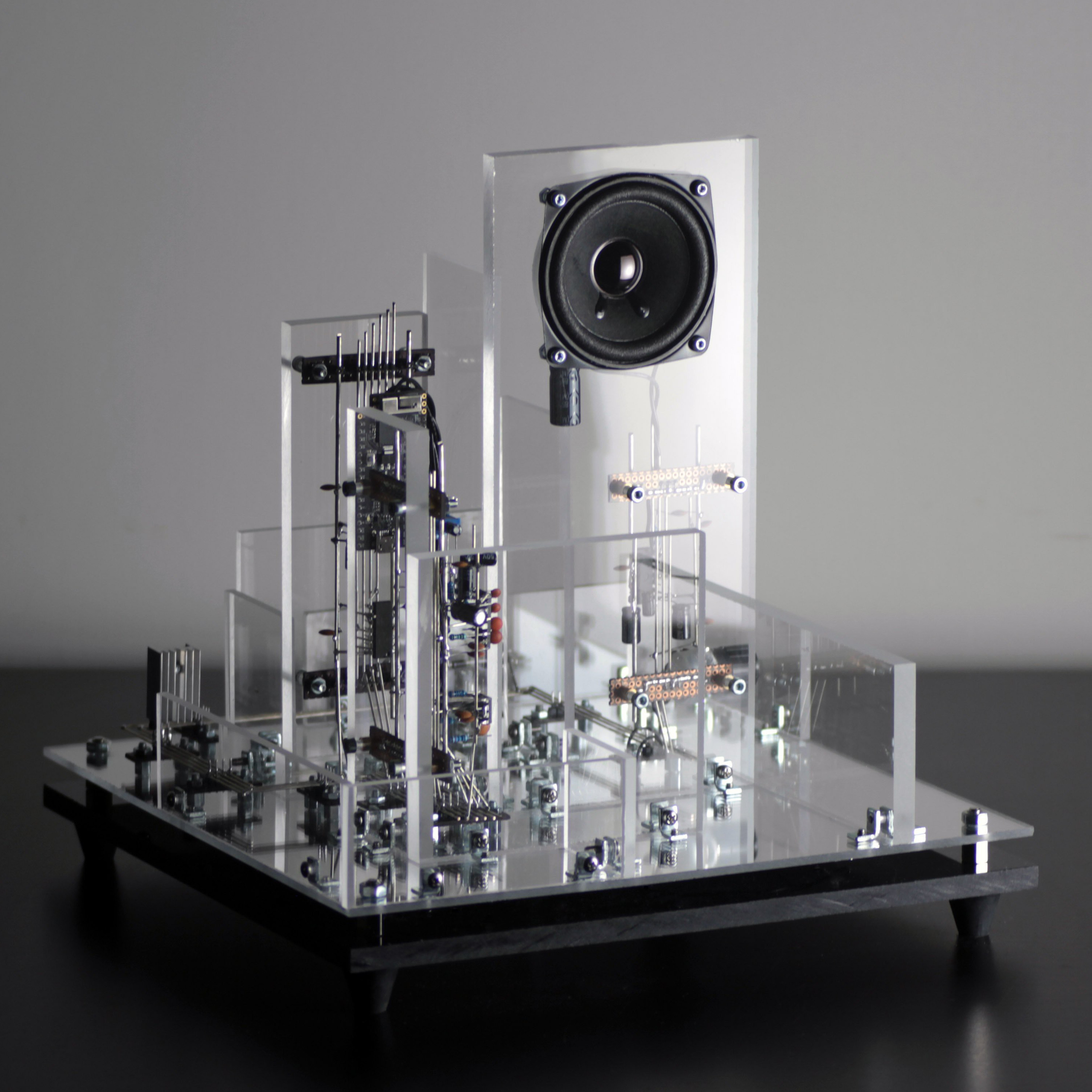This detailed photographic image, set indoors, captures a meticulously crafted engineering project that looks like a sophisticated model of an integrated circuit board. The construction features a black base supported by four feet, with a silver platform mounted atop it. Rising approximately 18 inches from the base, multiple metal rods (five in total) protrude vertically, and interspersed among these rods are black circuit boards. These circuit boards, connected by numerous small metal pieces and bolts, contribute to the intricate assembly that epitomizes electrical engineering.

In the background, there is a prominent white-framed speaker with a black circular speaker embedded and screwed into the top of the frame, suggesting the model may be part of a larger electronics project possibly related to audio equipment or a computer. The scene is set on what appears to be an engineering workbench, featuring miscellaneous metal and plastic components, indicative of an ongoing technical endeavor. The table is black, contrasting with the gray background, further emphasizing the functional and industrial nature of the setting. The entire image is devoid of any text, focusing solely on the detailed hardware and assembly process.